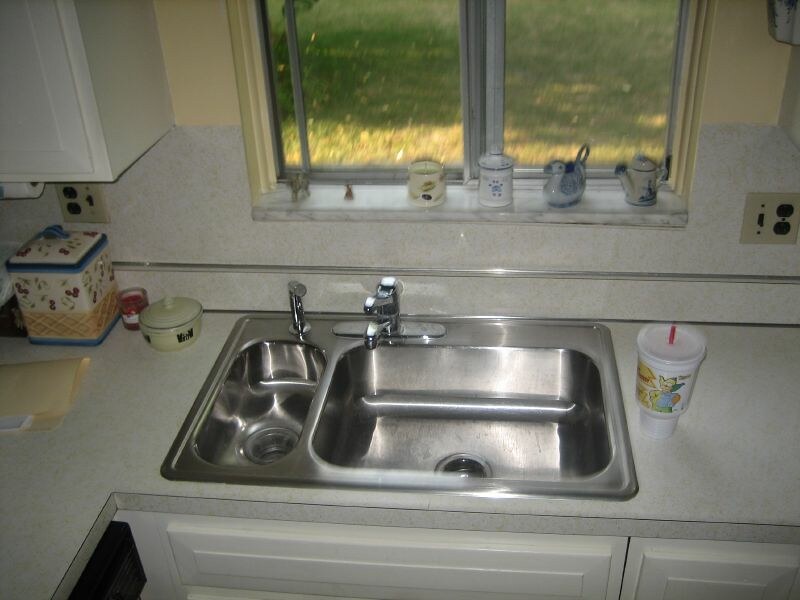This image showcases a detailed view of a kitchen, with the primary focus on a stainless steel sink embedded in a light gray countertop. The sink is an intricate structure with a large square basin on the right and a smaller, shallow section on the left, both featuring their own drains. The smaller left section appears to be a rinse station or possibly dedicated to a garbage disposal unit, complete with a pull-out spray nozzle, while the larger right basin has a traditional chrome faucet.

The counter surrounding the sink is white laminate, and directly behind the sink, there's a windowsill adorned with various porcelain items. In the scene, a plastic takeout beverage container with a red straw is prominently placed, along with a white cookie jar accented with blue and tan, and another treat jar which could be for a pet.

Below the counter are light gray drawers and cabinetry. Further details include a manila envelope filled with papers lying flat on the counter, a paper towel dispenser mounted under the cabinet, and a light switch paired with electrical outlets, all situated near a beige bracket.

In the upper left portion of the image, we see part of a white cabinet, and on the gray wall to the right, there’s a window with some grass visible in the background. This comprehensive setup gives a warm, functional, and slightly eclectic feel to the kitchen space.